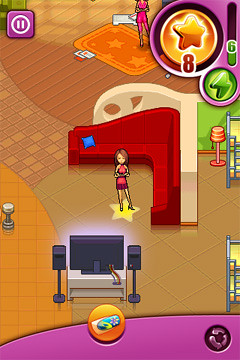The image depicts a vibrant, animated video game scene resembling the art style of The Sims. At the center is a female avatar, distinguishable by her red dress and short brown hair swept to the side. She stands on a yellow star, marking her as the player-controlled character. The room is richly detailed, featuring varied flooring—tile and wood—and includes a right-angle red sectional couch behind her. In front of the avatar is a large TV screen with surround sound speakers, which she appears to be watching. The background has an amber hue and an orange carpet adorned with stars. In the top right corner of the screen, a gold star with the number 8 and a green lightning bolt suggest game-related indicators or achievements. Additional elements include a pause button in the upper left corner and a woman in a pink pantsuit standing on the orange carpet. The room design includes steps and possibly a boutique area to the right, hinting at a complex in-game environment.